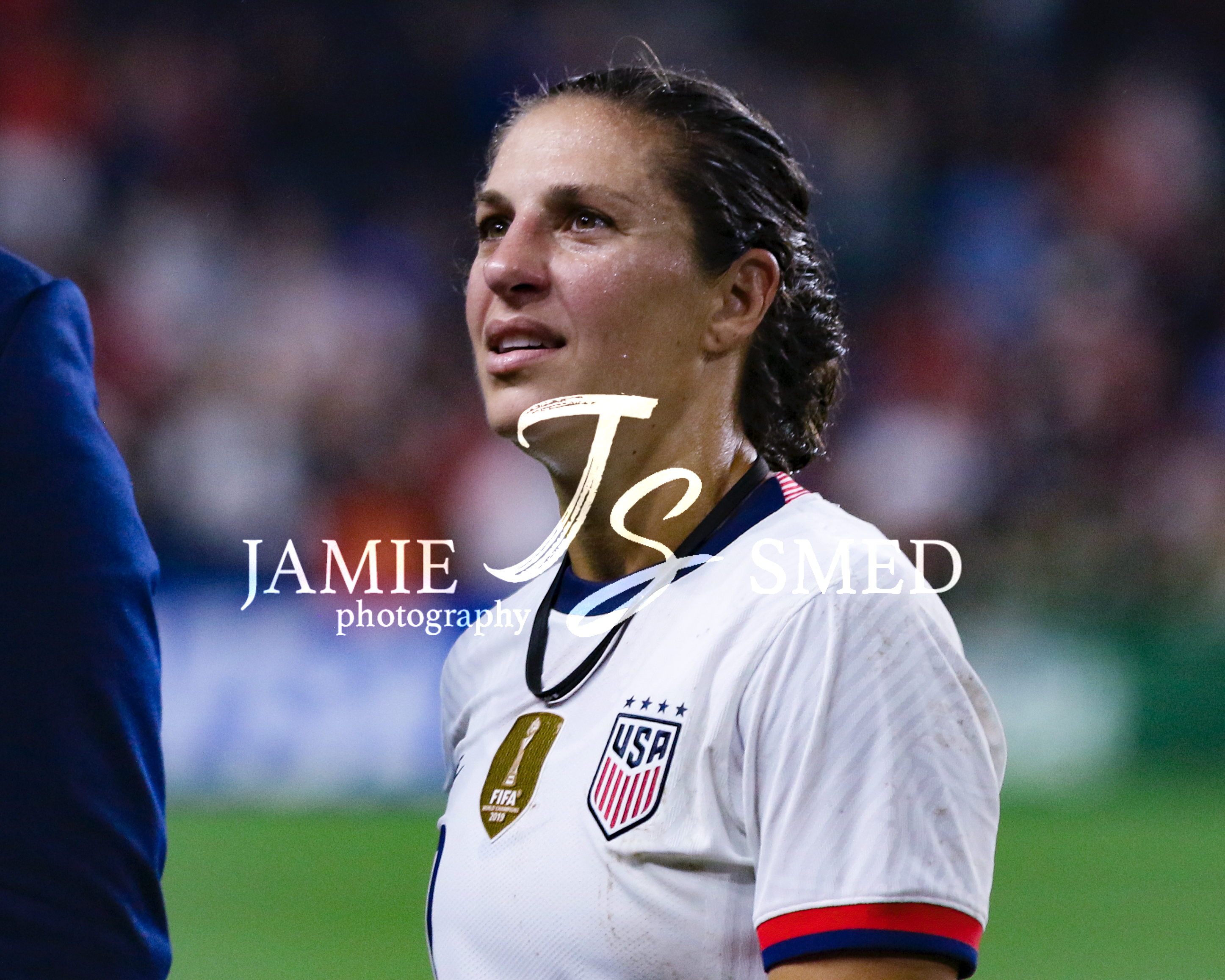This color photograph captures a close-up of a female athlete, a white woman with long dark hair, wearing a white Women's USA soccer jersey. The jersey is adorned with the logo "USA" in blue letters, accentuated by red stripes underneath. On the chest, slightly off-center towards the middle, there is an olive-green FIFA badge with white lettering, which seems to indicate the year 2019. The short sleeves of the jersey feature red and blue stripes at the ends. Around her neck, she is wearing a black necklace. The background, though blurry, reveals a green grass field and an out-of-focus crowd, possibly spectators or fans in bleachers. Overlaying the image is white text that reads "Jamie Smedd Photography," with the initials "JS" prominently displayed in the center. A person in a blue top is barely visible on the left edge of the image. The overall setting is well-lit, highlighting the details of the scene.